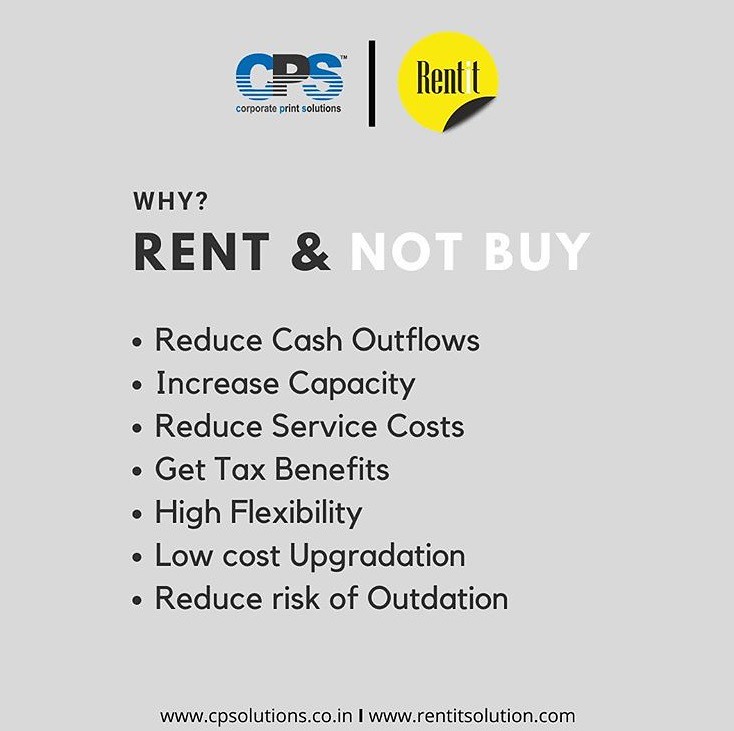The poster features a light blue-gray square at the top with the acronym "CPS" and a trademark symbol in the right corner. Below, it reads "Corporate Print Solutions" with a horizontal line underneath. Adjacent to this, there's a prominent yellow circle with the text "Rent It" written in black, where the "I" is white. The yellow circle has a slight bottom curve resembling a fingernail. Below the circle, the text "WHY RENT & NOT BUY" is displayed in all-capital letters, with "WHY RENT" in black and "NOT BUY" in white. The poster then lists several benefits in black text: "Reduce Cash Outflows," "Increase Capacity," "Reduce Service Costs," "Get Tax Benefits," "High Flexibility," "Low Cost Upgradation," and "Reduce Risk of Outdation." At the bottom, the small print lists two websites: "www.cpssolutions.co.in" and "www.rentitsolution.com."